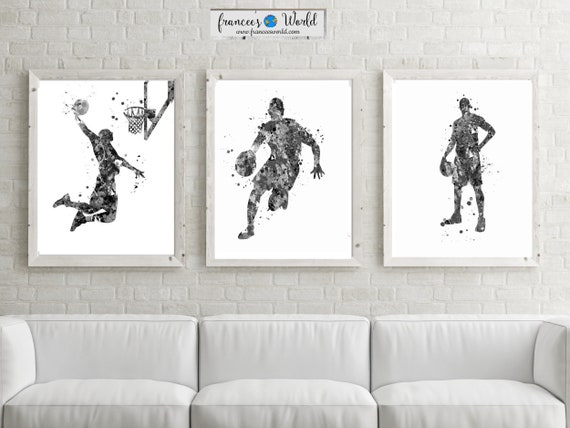In a tastefully decorated room with a white brick wall, a white three-cushion couch prominently fills the lower part of the frame. Above the couch, three evenly spaced, framed silhouettes of basketball players on white canvases depict dynamic scenes of the game. The left image features a player executing a slam dunk, with the hoop and backboard included, rendered in varying opacities of black ink spots. The center image displays a player dribbling down the court, and the right image captures a player standing with the ball. Each artwork is enclosed in a rustic, unfinished white wooden frame. Subtle but detailed, an inscription at the top reads 'France's World,' though the font makes it somewhat difficult to discern.